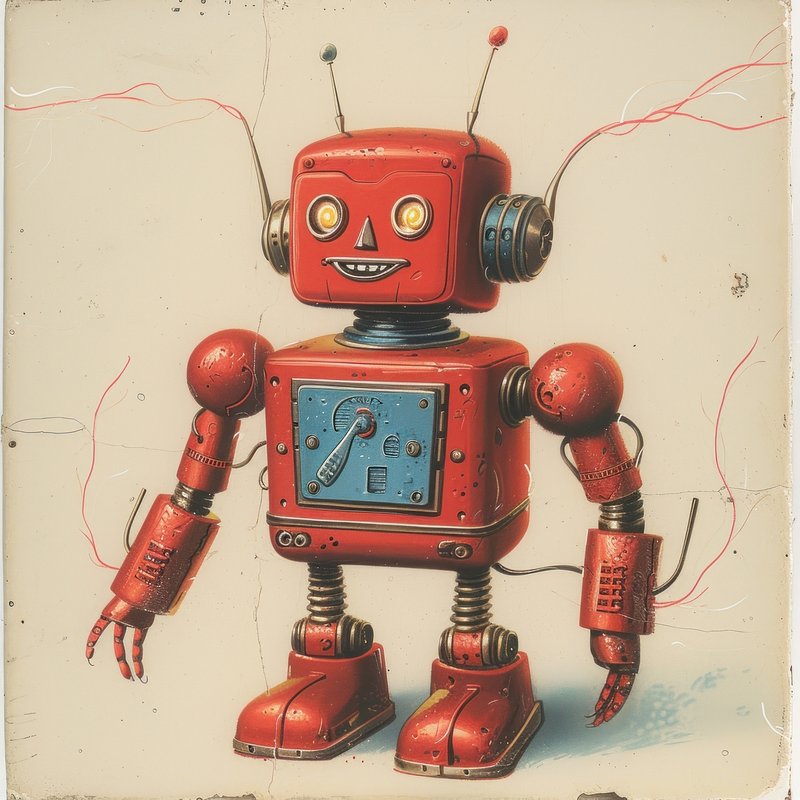The image depicts a retro-futuristic, cartoony red robot set against a tan background. This humanoid robot, designed with a cube-shaped head and body, has a distinctive old-fashioned appearance reminiscent of 1980s robotics. Its eyes are mesmerizing yellow spirals set in metal, and it features a triangular brass nose and a half-moon mouth displaying a fixed pseudo-smile with visible teeth. The robot’s "ears" look like metal headphone dials with red and white wires extending from them, along with two antennae sprouting from its head—one topped with a red knob and the other with a bluish or grayish knob.

The robot's neck looks like a black rubber joint, while its torso houses a blue door resembling a control panel with a turnable knob and textured, metal details. The limbs start with round ball-joint shoulders leading to segmented, cylindrical arms ending in three articulated fingers, and metal springs form its legs, giving the appearance of compressible coils. It stands on large, red, metal boots. Additional red wires protrude from its forearms and head, contributing to its intricate, cluttered design. The overall aesthetic combines bright red metal with blue and brass accents, rich in whimsical, retro charm.